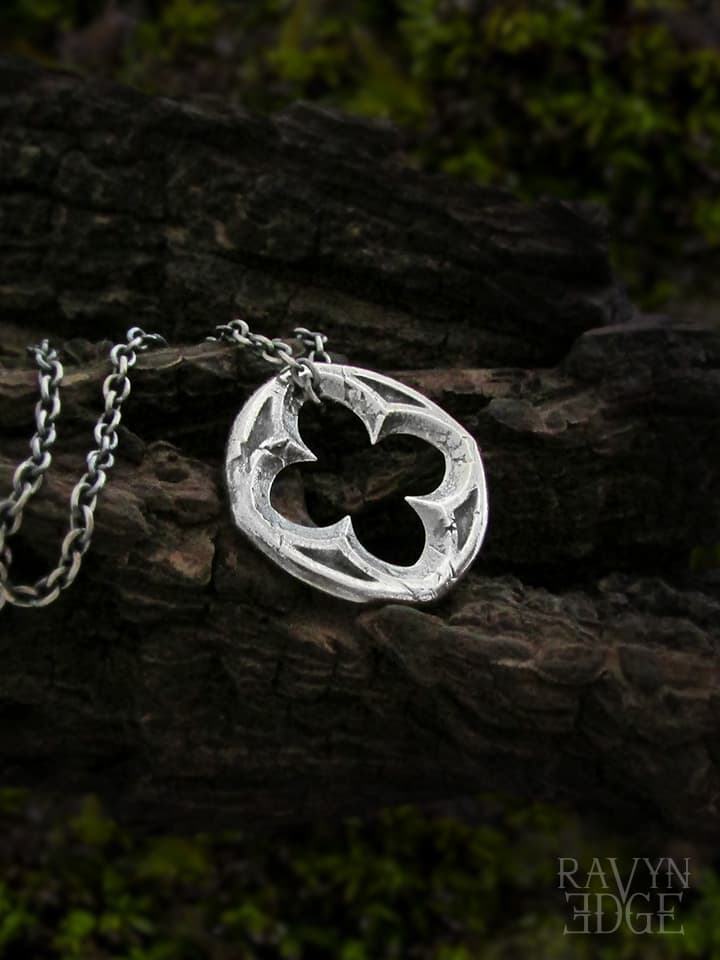The image showcases a piece of jewelry, specifically a circular silver pendant with an intricately etched pattern. The pendant features a cutout design resembling a cross with rounded protrusions, giving it an almost fleur-de-lis quality. It is adorned with a simple silver chain. This jewelry piece is set against a natural backdrop with dark green leaves and a tree branch on the ground, adding to the earthy, textured scene. The chain and pendant are prominently displayed atop the tree branch. In the bottom right corner of the image, there is a logo that reads "Ravyn Edge."